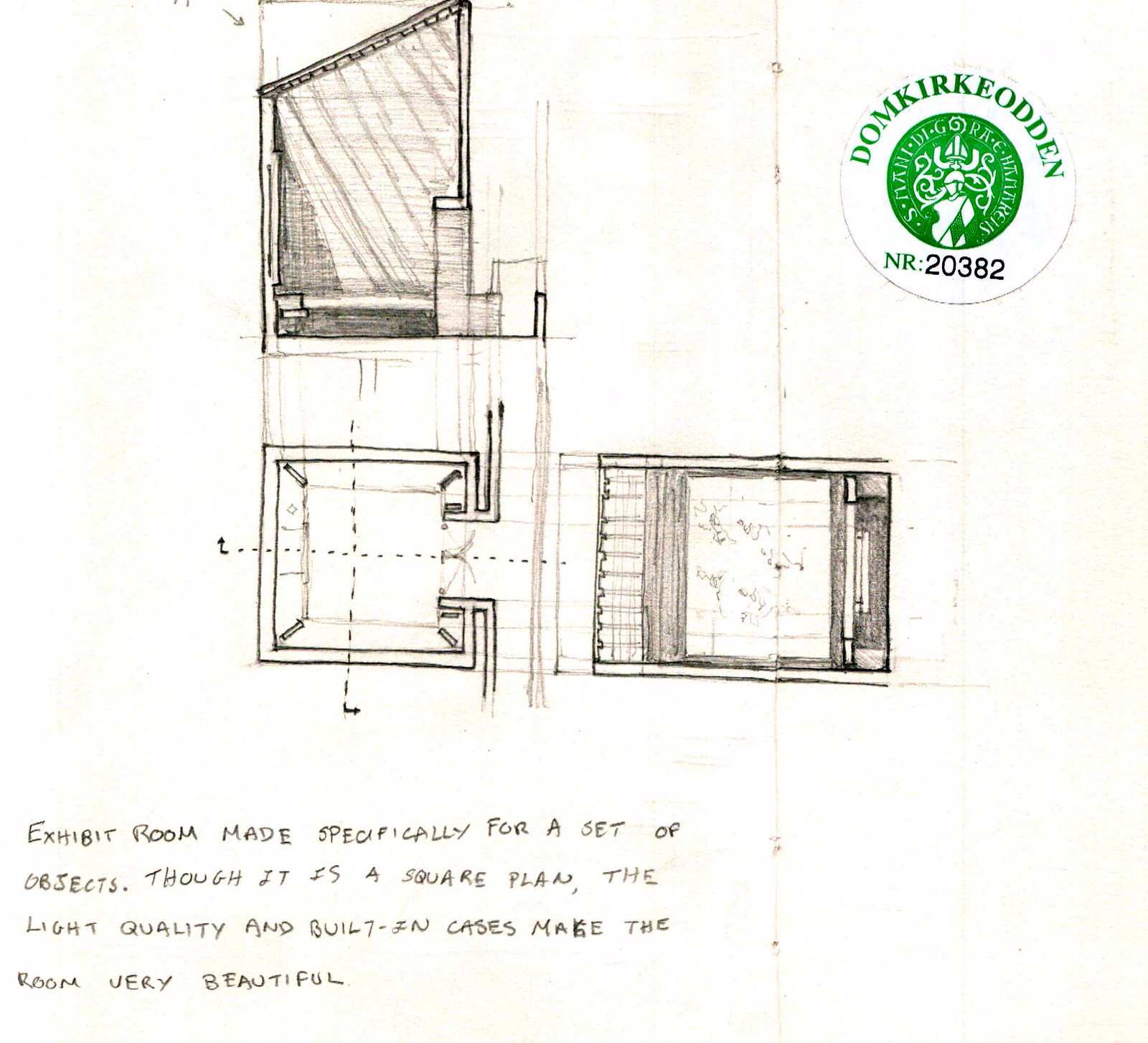This image is a detailed architectural drawing that appears to outline an exhibit room designed for displaying specific objects. The drawing is segmented into different sections: a top floor or room, a lower section with possible stairs and a hallway, and a third detailed drawing which is hard to interpret but might indicate another room or stair setup. Notably, each of these sections includes specific design elements like corridors, arrows, and pillars. 

At the top right corner of the drawing, there is a prominent green sticker with a central logo that appears to have a Celtic design, featuring a knight's helmet adorned with a cross and a flag. The label reads "Dom Kirkadon" at the top, followed by "NR; 20382" beneath the logo in black text. 

A key textual description below the diagrams mentions that the exhibit room, despite its square floor plan, boasts beautiful light quality and built-in display cases, enhancing its aesthetic appeal. The arrangement of these elements in the drawing suggests a meticulous approach to showcasing the space's functional and visual characteristics.